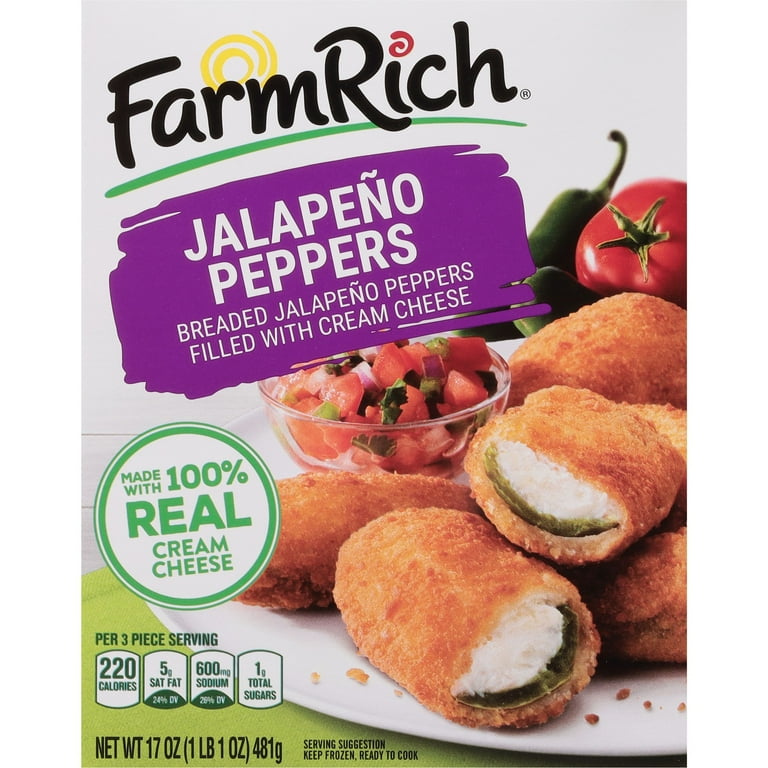This image depicts a box of Farm Rich Breaded Jalapeño Peppers filled with 100% real cream cheese, available for purchase at a grocery store. The Farm Rich logo, in black letters with a green underline and a sun situated above the "R" and "M," is prominently displayed at the top left. Below this logo, a purple splotch with white letters reads "Jalapeño Peppers." The packaging further details that the product consists of breaded jalapeño peppers filled with cream cheese. A green badge below emphasizes the use of 100% real cream cheese, with nutritional information indicating 220 calories per serving (three pieces). The image also shows the actual jalapeño peppers to the right, highlighting their breaded exterior and their creamy white and green interior. Accompanied by a clear bowl of freshly diced salsa in the center, composed of tomatoes and peppers, the visual also includes whole tomatoes and jalapeños in the background. Additional labeling on the package notes the product's net weight of 17 ounces and advises to keep it frozen until ready to cook. Nutritional details include 5 grams of saturated fat, 600 milligrams of sodium, and 1 gram of total sugars per serving.